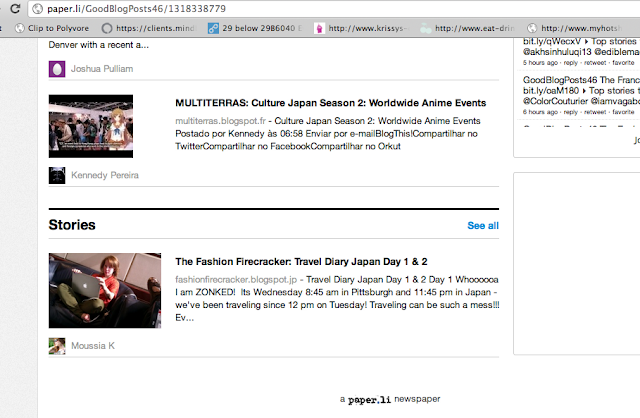A screenshot of a website is displayed with the URL bar indicating a blog post. Below the URL bar, several browser tabs are open, with titles such as "Clients" and "29 Below". The focused tab features an open webpage showing multiple articles. 

At the top, a partially visible article headline reads "Denver: A Recent Overview by Joshua Pullman". Below this, a clearly visible article titled “Multi-Terrain Culture in Japan: Season 2 Worldwide Anime Events” by Kennedy Arena is displayed. 

Under the main articles section, additional stories are listed including “The Fashion Firecracker” and “Travel Diary: Japan Day One and Two” by Musia. The website's design features gray font on a white background, which makes it somewhat difficult to read the text. There are various clickable pages allowing users to navigate through different articles on the site.